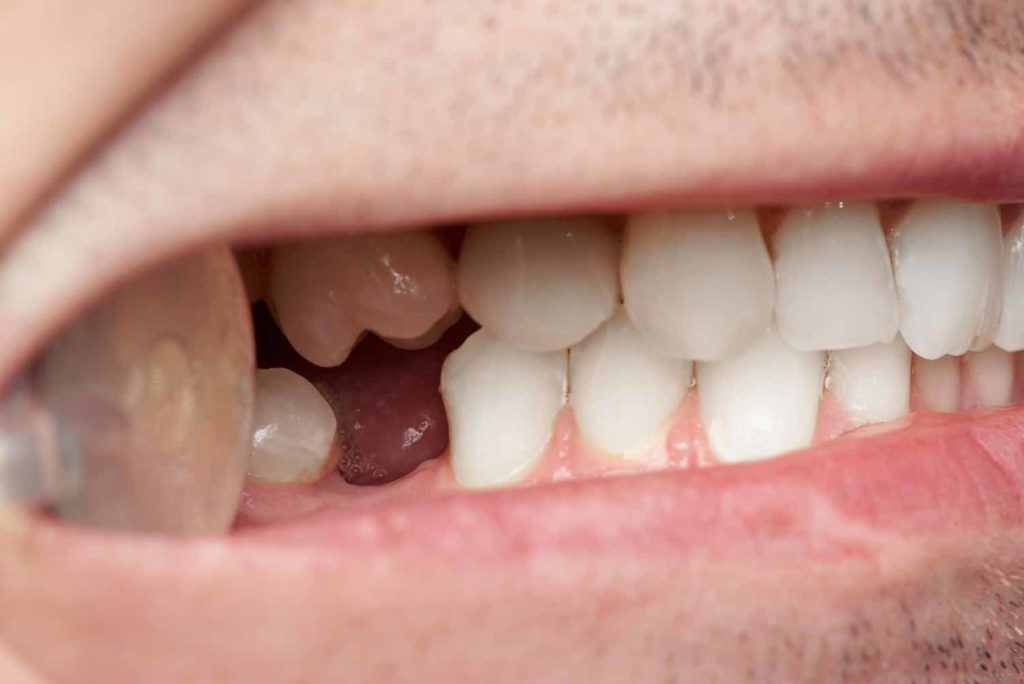The image is a close-up side view of someone's mouth, primarily focusing on the teeth and lips. The top and bottom rows of teeth are visible, with the top row showing five fairly white teeth, and the bottom row displaying seven teeth. There is a noticeable gap where a molar is missing in the bottom row, revealing pink gums and a red splotchy area at the back of the mouth. The teeth appear generally white, though darker and dingier towards the middle. The lips, which are pink, are being held open by a metal tool, possibly a dental retractor, situated on the left side of the image. Above and below the lips, there is evidence of stubble and shaved beard, with black and silver whiskers particularly visible on the lower right side. The person's gums seem healthy and you can glimpse the tongue and some saliva in the gap where the molar is missing.